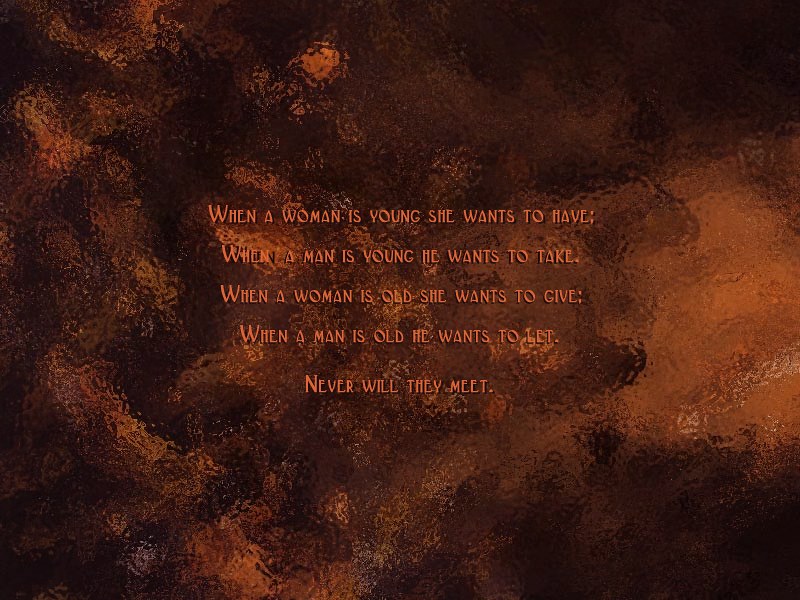The image features a digitally created, motivational card with a central quote that reads: "When a woman is young, she wants to have. When a man is young, he wants to take. When a woman is old, she wants to give. When a man is old, he wants to let. Never will they meet." The text is displayed in red capital letters, each line positioned horizontally, and enhanced with a black shadow drop. The background consists of a ripply effect resembling water splashes or disturbed water, with the look of stained glass. The colors transition in a palette of reds and browns, creating a smudged or rusty metallic appearance, with varying degrees of light and dark areas. The overall design combines these elements to emphasize the philosophical contrast between men's and women's perspectives at different life stages.